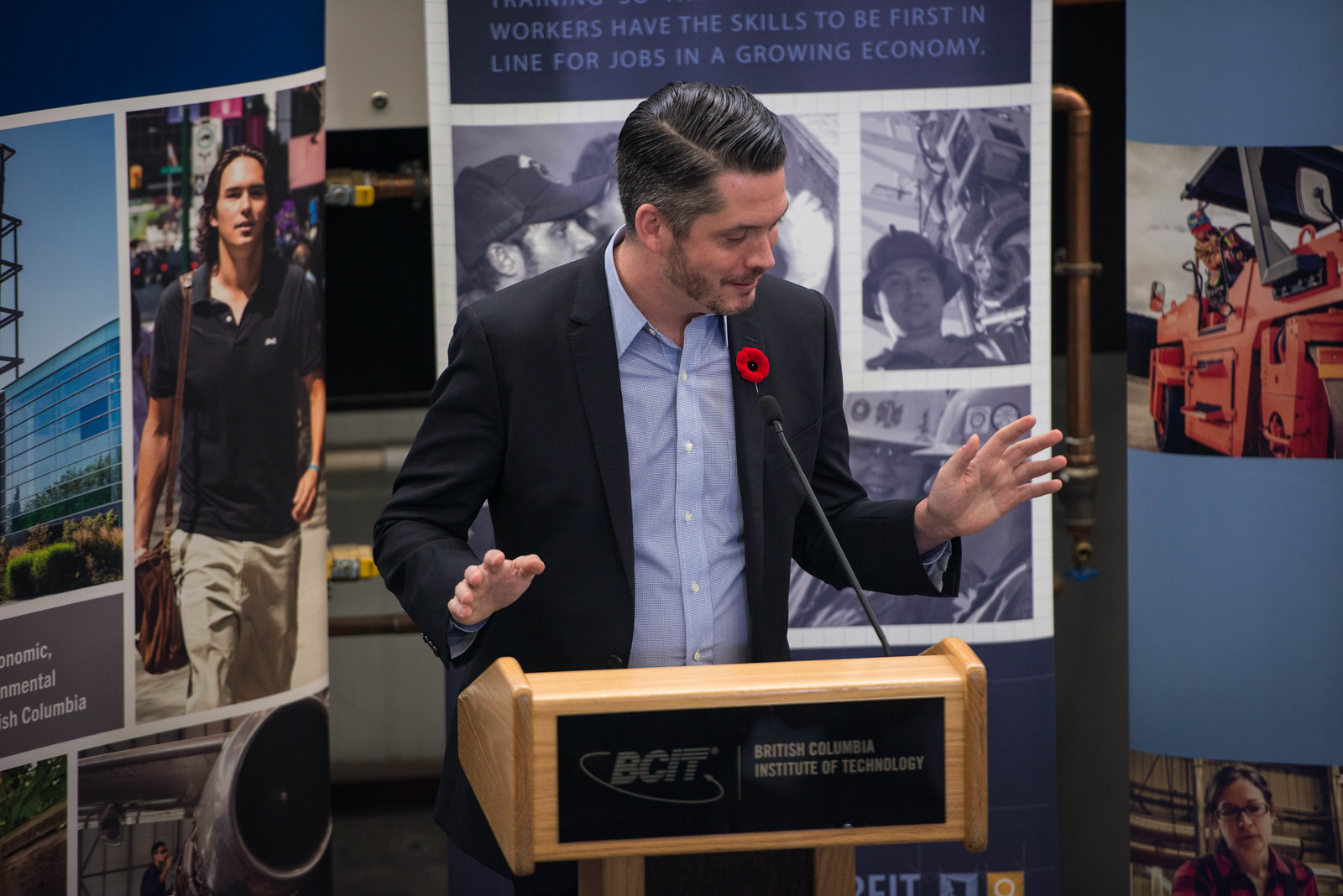In this indoor photograph, a man stands behind a wooden podium bearing the text "BCIT, British Columbia Institute of Technology," in gold lettering. Dressed in a blue button-down shirt and a dark-colored blazer, he has a red flower pinned to his coat and is speaking into a microphone. His hair is neatly combed and he gestures with both hands, emphasizing his speech. Behind him are three banners; the central banner features photographs and the words, "Workers have the skills to be first in line for jobs in a growing economy," while the other two banners display additional images with blue backgrounds but no visible text.